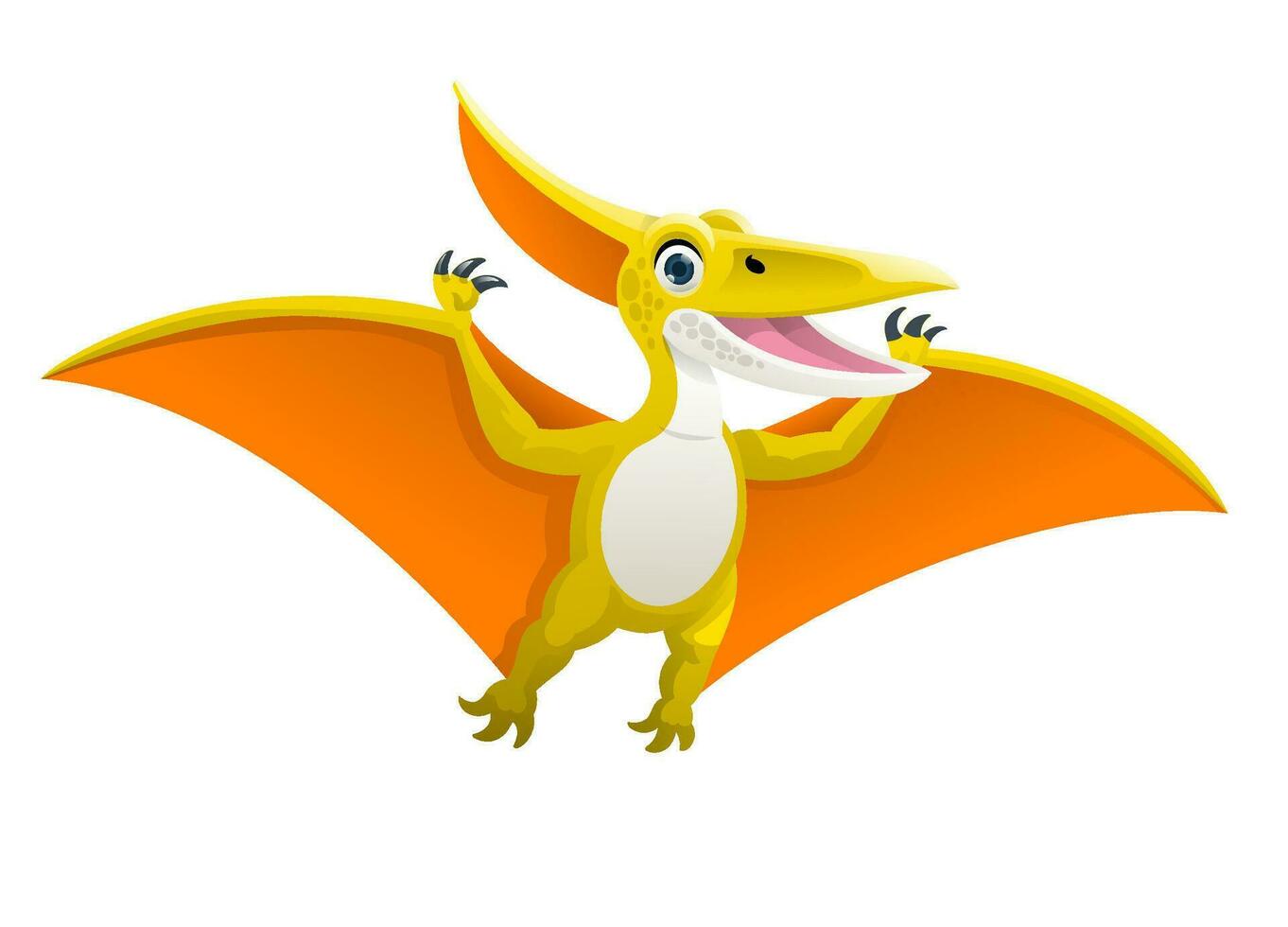This detailed, up-close image features a cheerful, animated cartoon character of a pterodactyl. The dinosaur's body is primarily yellow with a white chest, lower neck, and lower jaw. The inner sides of its wings are a dark orange, while the outer sides match its yellow body. It possesses a single, large orange crest on its head, shaped like a moon's crescent, and a small black nostril. The character's eyes are animated with a solid white base and black pupils, exuding a joyful expression. The pterodactyl's beak-like mouth is open, revealing a pink tongue inside, indicating it is smiling. It has three black claws on each hand, and its feet, also yellow, mirror this pattern. The image captures the pterodactyl in mid-flight, with its arms raised and body oriented towards the viewer, giving a sense of movement and excitement. The design's simplicity and bright colors, combined with minimal shadowing and scale detailing, suggest it is targeted towards young children. The lack of a detailed background focuses attention on the happy and vibrant character.